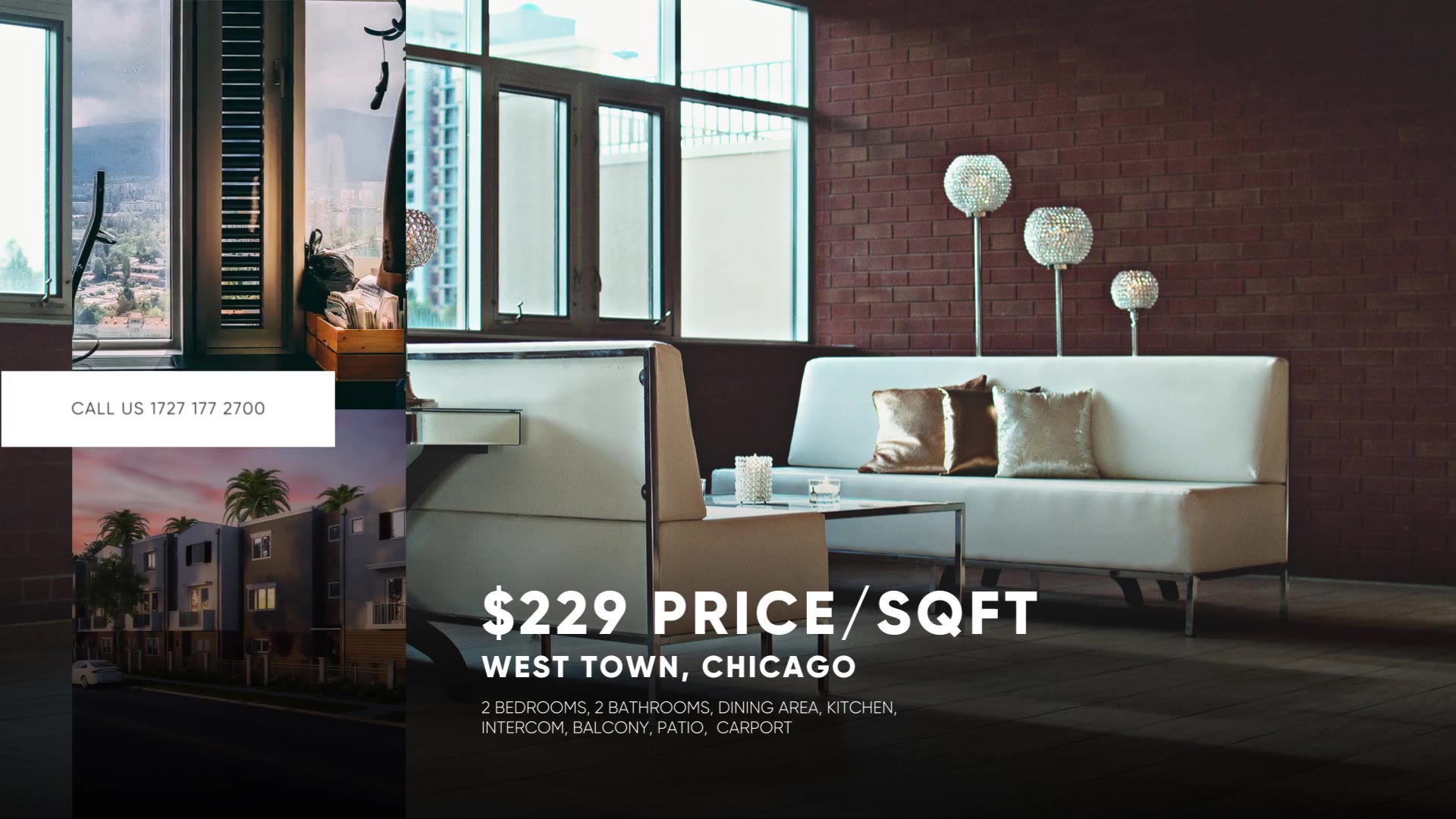A screenshot of a vibrant advertisement showcases a visually striking collage of architectural images paired with informational text. On the left side, two smaller, stacked square images grab attention. The top image presents an inviting interior scene featuring a couple of windows revealing a breathtaking view of a distant mountain. Below it is an exterior shot of an elegant, modern three-story apartment building. The building's base is crafted from brick, while the upper stories are constructed from wood or a similar material, all beautifully set against a twilight sky transitioning from pink to purple, complemented by the silhouettes of palm trees.

Centrally placed between these two images is a prominent white box displaying contact information: "Call us, 1727-177-2700."

Occupying the right three-quarters of the frame is a large, inviting interior image. A striking red brick wall lines the right, contrasting with a series of windows on the left that emit a subtle blue hue. The room's centerpiece features two pristine white couches positioned around a glass coffee table, evoking a sense of modern elegance. Adjacent to the brick wall, three unique lamps designed with a disco ball aesthetic add a touch of quirky sophistication. At the bottom left of this large image, white text details the property's specifics: "$229 price per square foot, West Town, Chicago. Two bedrooms, two bathrooms, dining area, kitchen, intercom, balcony, patio, carport."